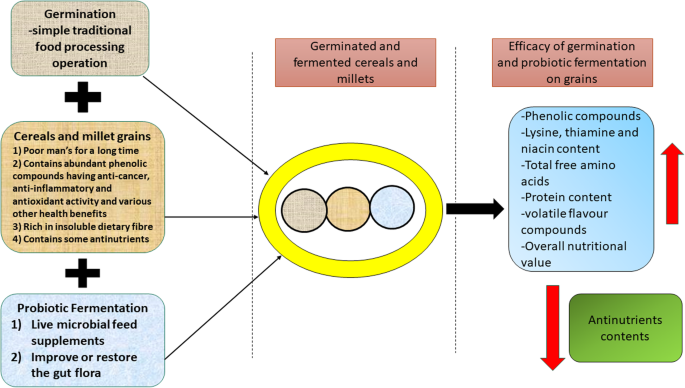The image is a detailed flowchart illustrating the germination and probiotic fermentation of cereals and millet grains, organized into three main sections. 

Starting on the left, the first column features three vertically arranged rectangles with rounded edges. The top rectangle, light gray, contains the text "Germination: Simple Traditional Food Processing Operation." Below it, marked by a plus sign (+), is another light brown rectangle labeled "Cereals and Millet Grains" with four talking points underneath. The bottom rectangle with a blue background reads "Probiotic Fermentation" and is accompanied by two bold points. Each section has a black line converging towards the center of the chart.

In the middle column, a central yellow oval with a white background contains three nested circles in light blue, gray, and brown. Above this oval, there's a light purple rectangle labeled "Germinated and Fermented Cereals and Millets." 

The third column on the right features three rectangles with rounded edges and different background colors. The top rectangle, light purple, states "Efficiency of Germination and Probiotic Fermentation on Grain." In the middle, a blue rectangle lists "Vanilla Compounds, Lysine, Thiamine, Niacin Content, Total Free Amino Acids, Protein Content, Volatile Flavor Compounds, Overall Nutritional Value," with a red arrow pointing downward and another pointing upward. The bottom green rectangle notes "Anti-nutrient Contents."

The arrows and the color codes (light gray, light brown, light blue) guide through the logical progression of germination and fermentation effects on cereals and millets, highlighting the nutritional outcomes and efficiency metrics. The red arrows emphasize key transitions between the sections.